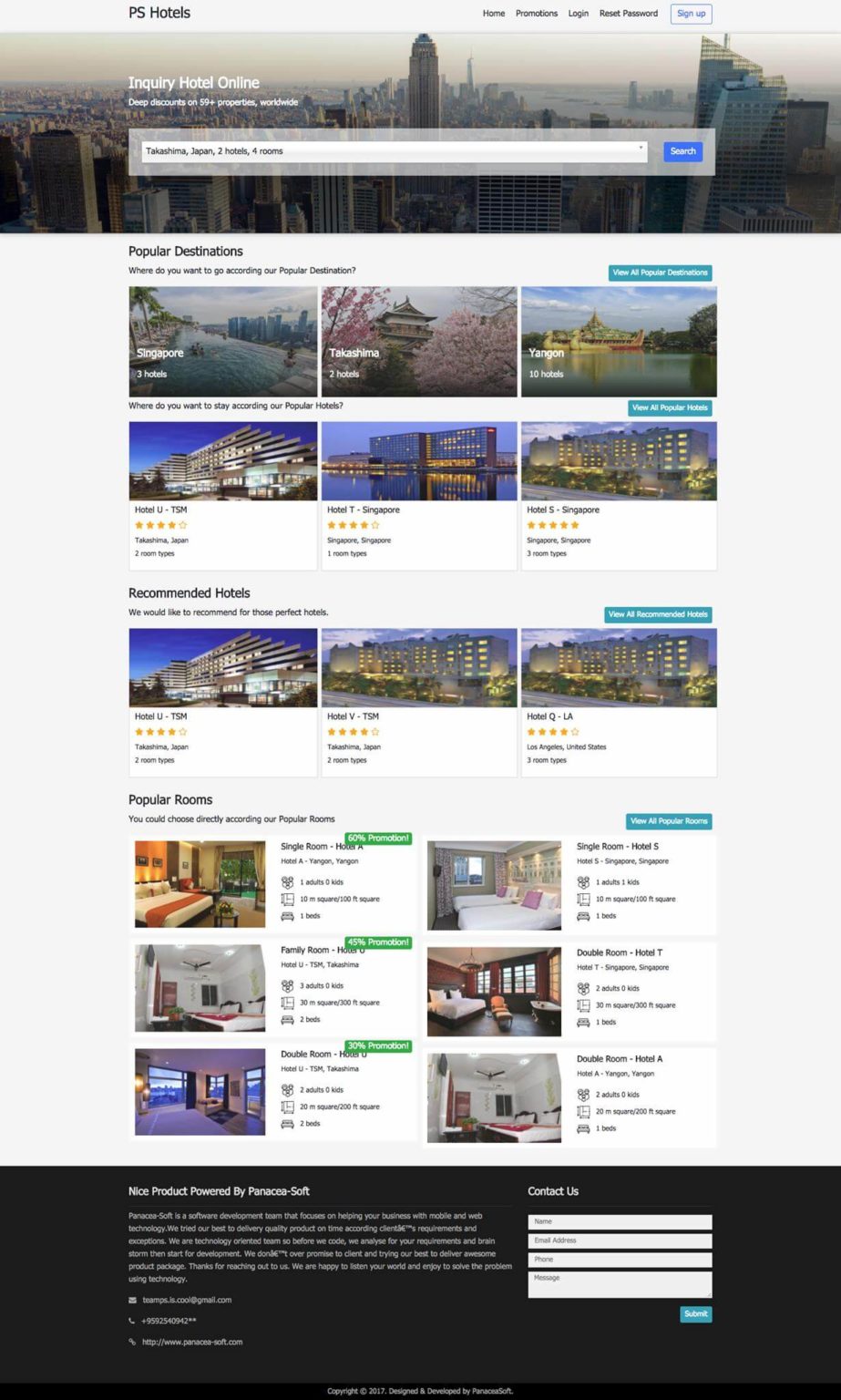This image showcases the complete webpage of the P.S. Hotels website. The page features a light gray banner at the top prominently displaying "P.S. Hotels." Along the banner, there is a navigation menu with the word "Home" clearly visible and possibly three to four additional menu items, although their exact text is hard to discern. There is also a rectangular sign-up box with some text inside it.

Below the banner, the webpage integrates a backdrop of a cityscape with the text "inquiry hold online." Directly underneath this, there is another gray banner containing a search bar. The search bar has a white rectangular field with labels or information on the left side and a blue "Search" button on the right.

Following the search section, the page highlights "Popular Destinations," featuring three prominent images. The central image appears to be an oriental scene, while the first one seems to depict the coastline of Singapore. The remaining images are not easily identifiable. Below these, there's another series of three images, each accompanied by ratings.

Further down, the site presents "Recommended Hotels," displaying three images along with their respective ratings. This section is followed by "Popular Rooms," which includes six images. Among these, three have green banners, while one boasts a blue banner.

At the very bottom of the page, there is a "Contact Us" section, providing a final point of engagement for visitors.